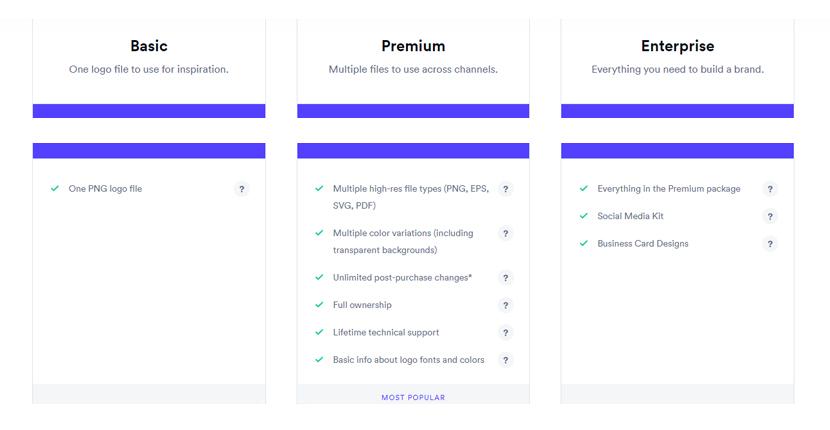A color, computer-generated landscape image depicts what appears to be a screenshot from a website on a laptop or a computer display. The screenshot showcases a comparative chart of three different product purchasing tiers: Basic, Premium, and Enterprise. Each tier offers varying levels of service and is presumably priced progressively higher, although specific prices are not shown. 

The **Basic** tier includes a single PNG format logo file intended for basic use or inspiration. 

The **Premium** tier offers a more comprehensive package, providing multiple high-resolution logo files in various formats such as PNG, EPS, SVG, and PDF. It also includes multiple color variations, transparent backgrounds, unlimited post-purchase changes, full ownership rights, lifetime technical support, and detailed information about the logo's fonts and colors. 

At the highest level, the **Enterprise** tier encompasses all benefits of the Premium package and adds a social media kit along with business card designs, effectively equipping users with the complete toolkit needed to build a robust brand presence. Additional capabilities and services are included as one progresses from Basic to Enterprise, emphasizing the value increment at each tier.